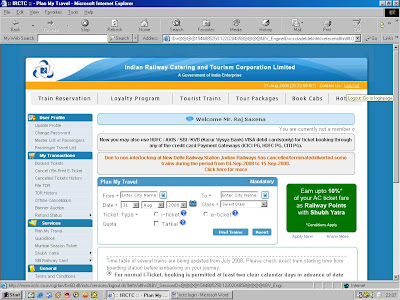This image captures a screenshot of a computer displaying the Indian Railway Catering and Tourism Corporation Limited (IRCTC) website. The interface features a standard computer screen layout, with a gray top bar populated with various icons typical of a web browser. 

Dominating the screen, the middle section of the webpage is enveloped in a royal blue background, prominently presenting a white rectangle with the text "Indian Railway Catering and Tourism Corporation Limited" and the tagline "A Government of India Enterprise."

Beneath this header, a golden yellow stripe runs horizontally across the page, serving as a navigation bar. This bar includes clickable options labeled "Train Reservation," "Loyalty Program," "Tourist Trains," "Tour Packages," and "Book Cabs." A partially obscured option that begins with "HOT" suggests links to "Hotels."

Further down, a personalized greeting, "Welcome Mr. Rajasarva," is displayed. Underneath this greeting are two elongated rectangular buttons, followed by another rectangle labeled "Plan My Travel." A highlighted message indicates an opportunity to "earn up to 10% of your AC ticket fare as railway points with Shabda Yatra."

Additional clickable sections populate the page, offering users various interactive features and services designed to facilitate travel planning and booking through the IRCTC platform.